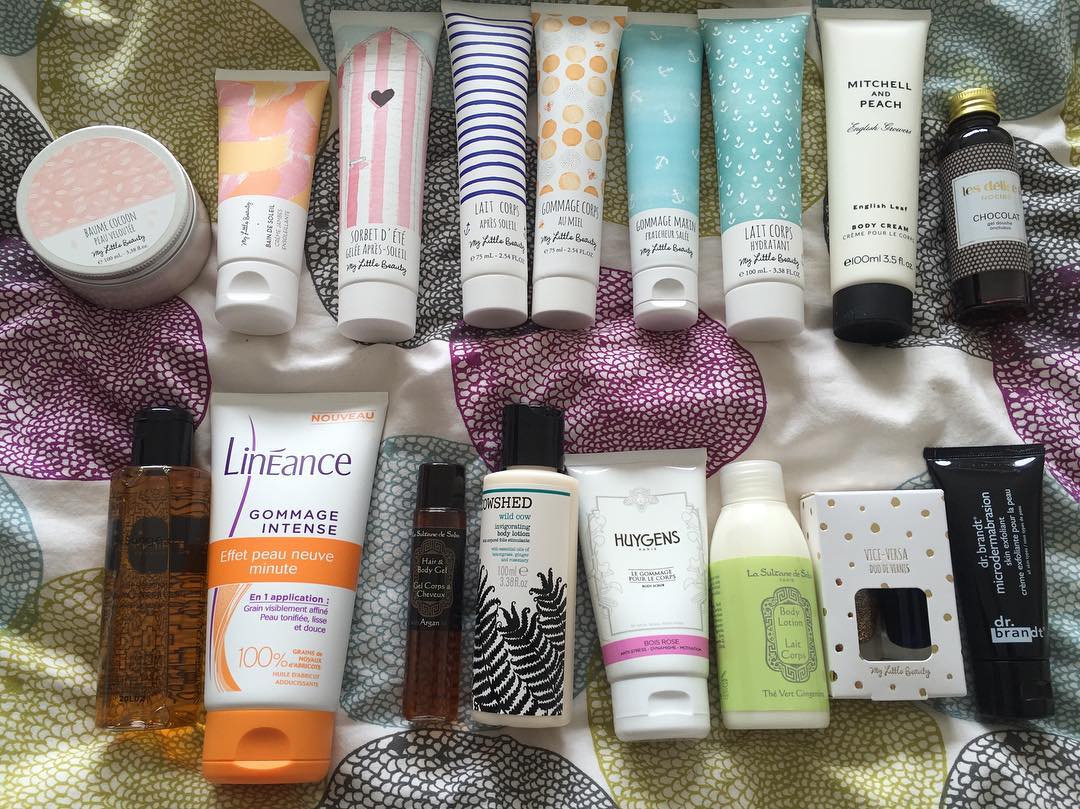This is a detailed horizontal photograph showcasing a diverse collection of creams and beauty products arranged meticulously on an intricately patterned fabric background. The fabric spans the entire frame and features a striking design composed of large circular motifs filled with numerous elongated ovals. The central circle is a deep wine color, bordering on magenta, while the surrounding circles vary in shades of gray, black, and vibrant yellow-green.

The beauty products are organized into two horizontal rows. The top row occupies the upper third of the image, with each item placed vertically from left to right. The bottom row similarly places items in the lower third of the image.

In the top row:
1. A circular tin can with a tin lid, adorned with a sticker. The sticker features a light pink semicircle and black text on a white background.
2. Seven tubes of various sizes and designs:
   - The first tube is short, slightly larger than the tin can, with a white flip-top cap. The tube features white, pink, yellow, and orange colors.
   - The second tube is taller, with pink and white stripes and a black heart on one of the pink stripes.
   - The third tube is white with horizontal navy blue lines.
   - The fourth tube has a white background with orange and peach circles.
   - The fifth tube is turquoise with small white anchors.
   - The sixth tube is also turquoise with a white intricate design.
   - The seventh tube is primarily white with black text and a black flip-top cap.
3. A small brown glass jar with a white sticker, a brown background, a decorative design, and a gold lid.

In the bottom row:
1. A clear plastic jar with a black lid, positioned on the left side.
2. A large orange tube labeled "Lineance," featuring an orange band with white font and an orange cap.
3. A small brown bottle.
4. An off-white container with black plant designs and a black cap.
5. A white tube labeled "HUYGENS" in black font, with a pink band near the bottom.
6. A white bottle of cream with an olive green sticker around it.
7. A white cardboard box with brown polka dots, featuring a window in the bottom half (contents not visible).
8. A black tube with white font.

This detailed arrangement provides a visual feast, perfectly blending vibrant beauty products with an eye-catching patterned backdrop.